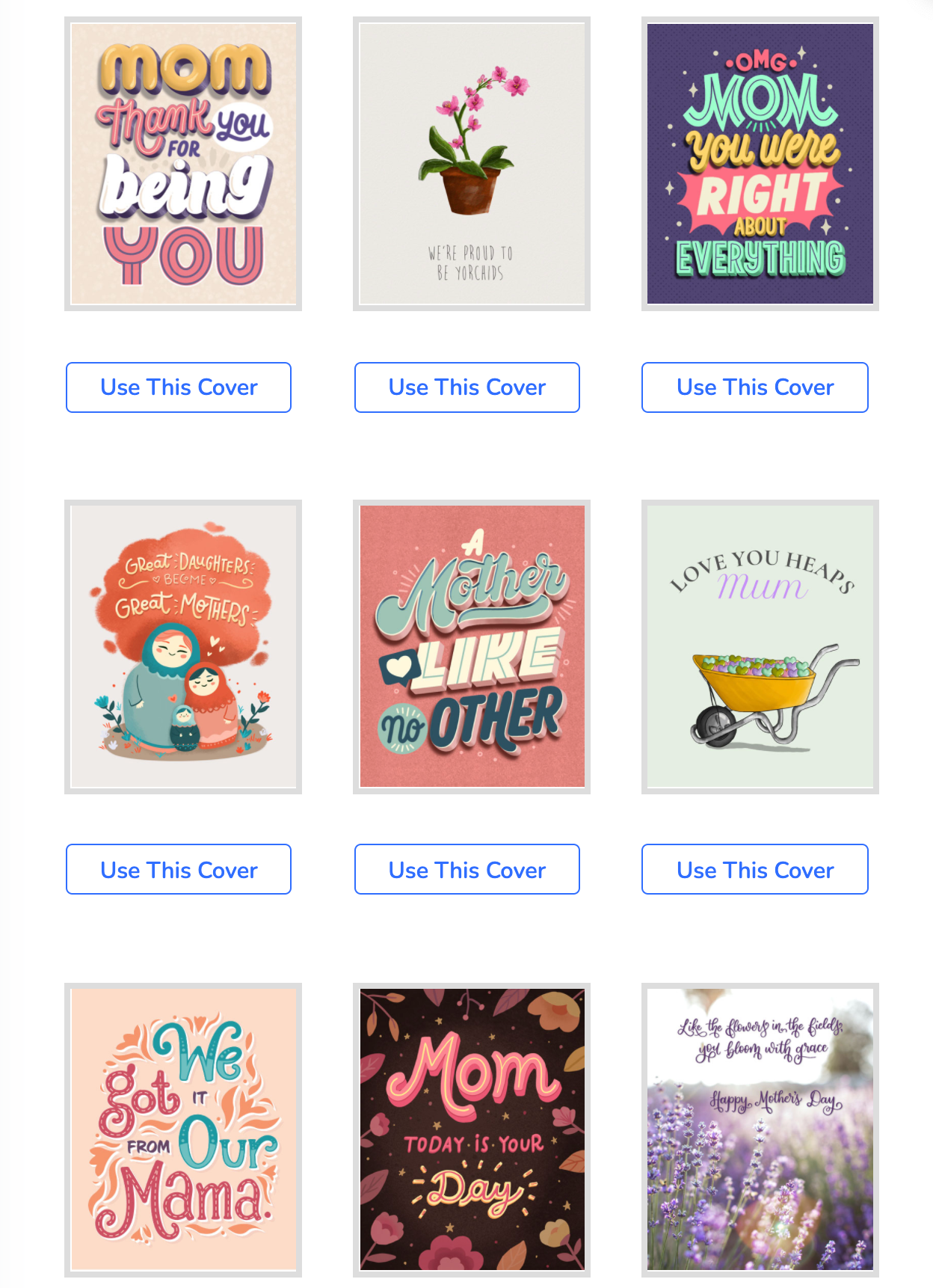A selection of nine beautifully designed Mother's Day greeting cards arranged in three rows of three on a white background. The top two rows each feature a blue-outlined rectangle beneath each card, labeled "use of cover" in blue, indicating a possible placeholder or template. The bottom row does not have these rectangles, suggesting an incomplete or cropped view.

Zooming into the details, the cards are as follows from left to right, top to bottom:

1. A heartfelt card with the message, "Mom, thank you for being you," expressing appreciation for a mother's unique role.
2. An adorable illustration of a little pink plant in a brown pot, featuring a playful and quirky message, "We're proud to be your kids."
3. A humorous and relatable card stating, "OMG, Mom, you were right about everything," recognizing a mother's wisdom.
4. An artistic design of three Russian nesting dolls with the message, "Great daughters become great mothers," celebrating the generational bond.
5. A sentimental card that reads, "Mom, a mother, love like no other," honoring the unparalleled love of a mother.
6. A charming illustration of a yellow wheelbarrow filled with love hearts in various colors, accompanied by the text, "Love you heaps, Mom."
7. A playful nod to maternal influence with the message, "We got it from our Mama."
8. A simple yet meaningful card declaring, "Mom, today is your day," perfect for celebrating the special occasion.
9. An elegant design featuring lavender flowers with the poetic inscription, "Like the flowers in the field, you bloom with grace. Happy Mother's Day," written in a delicate, old-fashioned script.

These cards collectively offer a range of messages from humorous to heartfelt, perfect for expressing love and gratitude on Mother's Day.